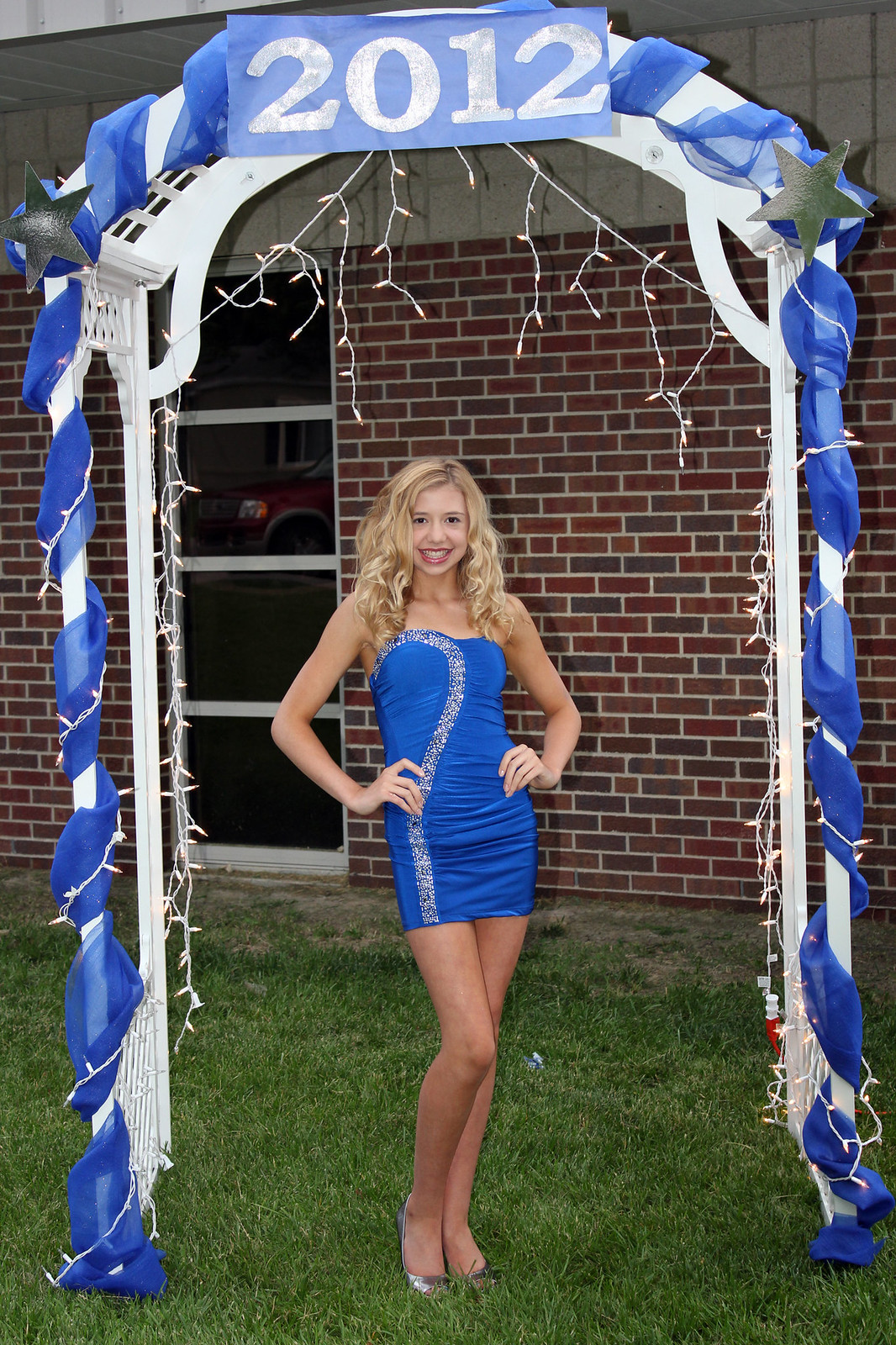This rectangular photograph captures a young girl, likely between 14 to 16 years old, posing elegantly under a white lattice garden arch adorned with blue gauze ribbons and possibly some Christmas-like strand lights. A prominent sign with a blue background and large white text displaying "2012" adorns the top of the arch, suggesting a special event, possibly prom or graduation. The girl stands confidently with her hands on her hips, showcasing her strapless short blue dress and silver high-heeled shoes. Her long blonde hair cascades in curls past her shoulders. The background features a brick wall punctuated by a vertical series of windows. In the third window up, the reflection of the front end of a red vehicle is visible. The ground beneath her feet is grassy, appearing slightly overgrown and in need of mowing.